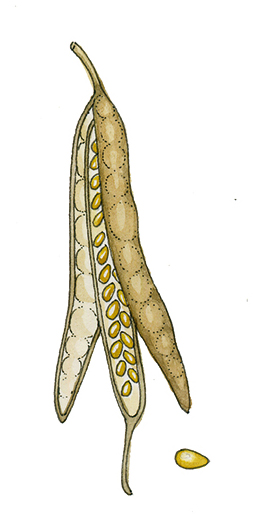This image is a detailed drawing of a cracked-open seed pod, possibly resembling a pea pod or some type of bean pod. The illustration is typical of what you might find in a textbook or an encyclopedia. The pod is oriented vertically and has a brownish-green hue, suggesting it might be dried out. The pod is divided into three longitudinal sections – the back, middle, and front. As it splits open toward the bottom, it reveals numerous golden seeds arranged along the middle section. The exterior surface of the pod features a bubbled texture. Notably, one small seed has fallen out and is lying on the flat surface below the pod, along with an additional downward-pointing stem connected to the middle of the pod. The illustration highlights the intricate structure and detail of the pod, offering an educational view of its anatomy.